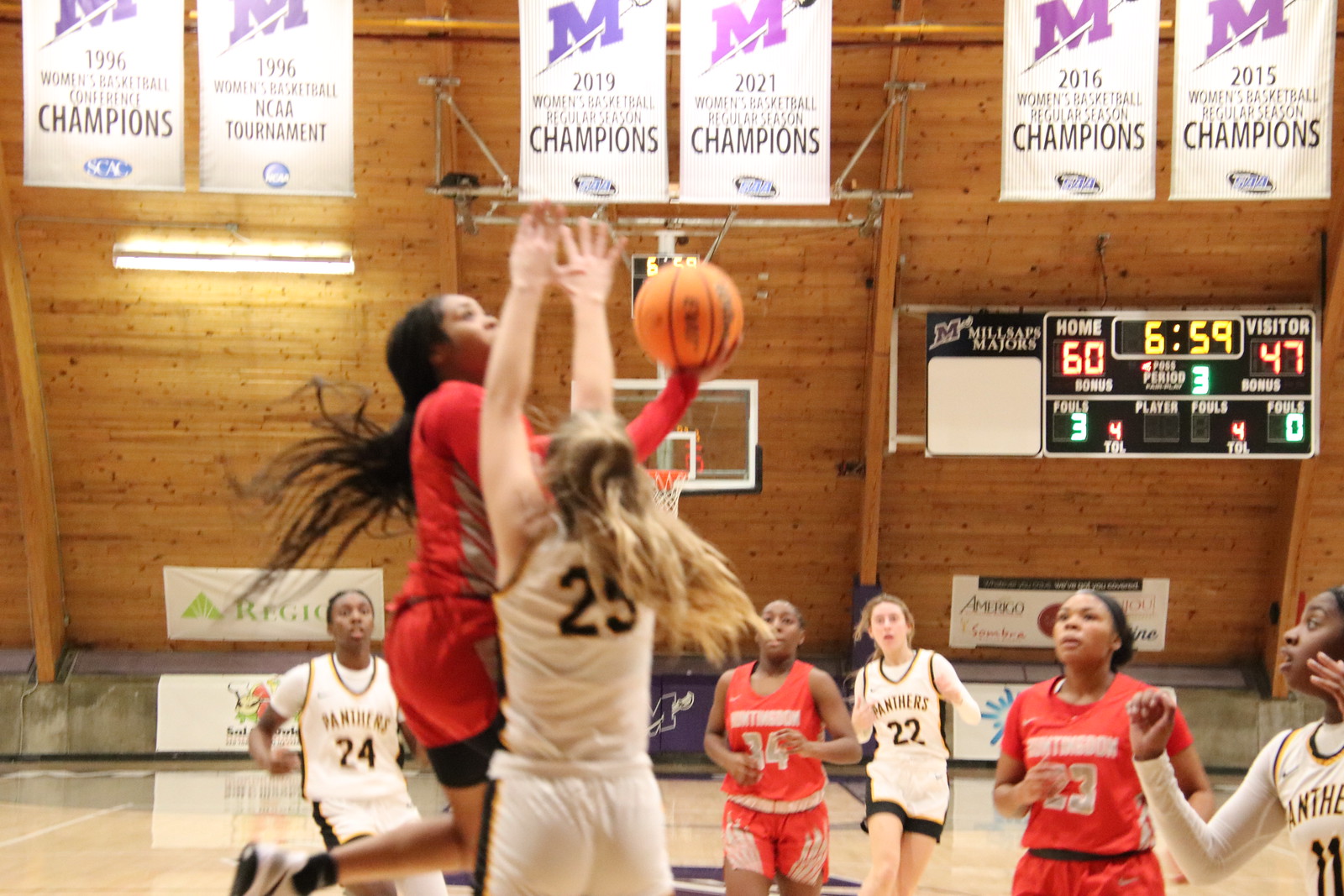This image is a color photograph of a live-action women's basketball game, likely at the high school or college level, taken inside a gymnasium. In the foreground, a player in a red uniform, a Black girl with long black hair, is seen jumping higher than her opponent, holding the basketball and attempting to score. Directly in front of her is a Caucasian girl with long blonde hair, wearing a white uniform numbered 25, who is also airborne with both hands raised in an effort to block the shot. 

In the background, five more players can be seen: two in red uniforms—both Black girls—and three in white uniforms, two of whom are Black girls with the other being Caucasian. The gymnasium features a ceiling adorned with six different banners marking championships, prominently displaying titles like "1996 Women's Basketball Conference Champions" and an "M" logo. Along the far wall, there is an electronic scoreboard showing the home team leading with a score of 60 to 47, with 6 minutes and 59 seconds left in the third period. The scoreboard also has various statistics, including fouls and tolls, and a section for player fouls, currently empty. Additionally, there are numerous advertisement banners from various companies lining the walls and borders of the court.